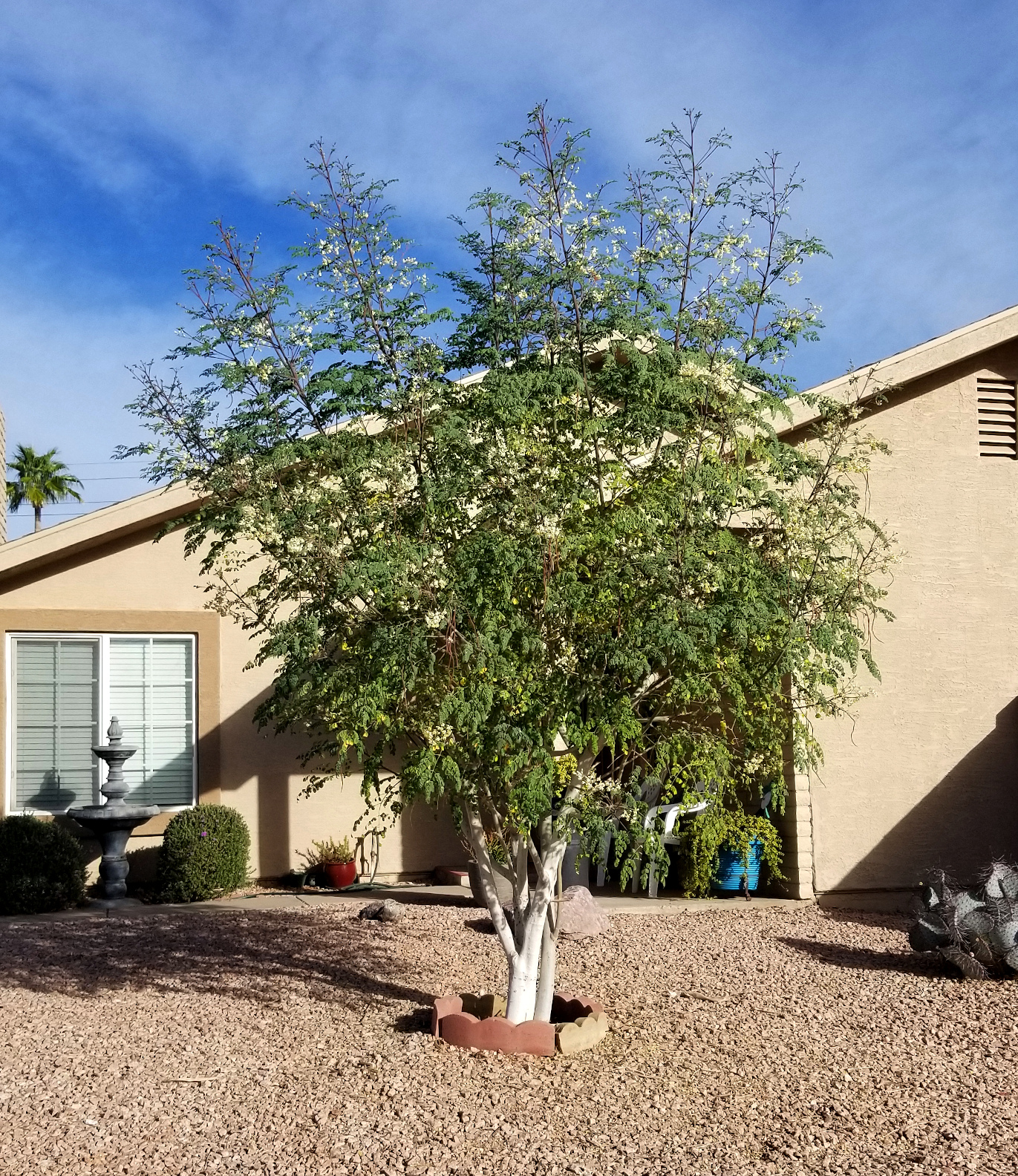This image captures the exterior of a beige stucco house, typical of southwestern or xeriscaped regions, under a clear, blue sky with wispy clouds. The yard features no grass, instead covered in tan rock and gravel. The focal point is a large tree with a striking white trunk and green leaves, adorned with white buds, which stands prominently in the center, flanked by a circular red clay protector around its base. To the left of the tree is a window adorned with neatly trimmed green bushes and a decorative water fountain. Nearby, the ground hosts a possible cactus plant, partially enveloped in shadow, adding to the desert ambiance. In the background, a distinctly silhouetted palm tree rises above the house, adding to the characteristic southwest landscaping. Additionally, a pair of white plastic chairs is visible in the yard, along with a blue pot containing another plant, further embellishing the scene.